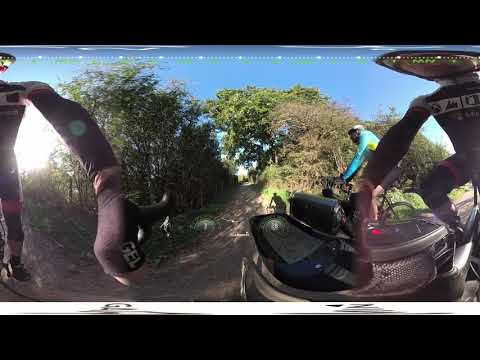The image captures a bright, daytime moment on a dirt bike trail surrounded by green trees and a clear blue sky. From the perspective of a bicyclist taking a selfie, the scene features three cyclists. The central figure in the foreground is dressed in all black with a matching helmet, and his thumb is visible to the side, pointing backward with a gloved hand that reads "G-E-L." Next to him, another cyclist is seated with one leg extended on the ground for balance, wearing black bike shorts, a turquoise shirt, and a helmet. Close by and riding towards the left side of the image is a third cyclist in a blue and yellow long-sleeved spandex shirt, also wearing a helmet. This cyclist appears in motion, contrasting with the other two who are stationary. The image also reveals some brush in the background, adding to the natural setting of the dirt path where the cyclists are captured.